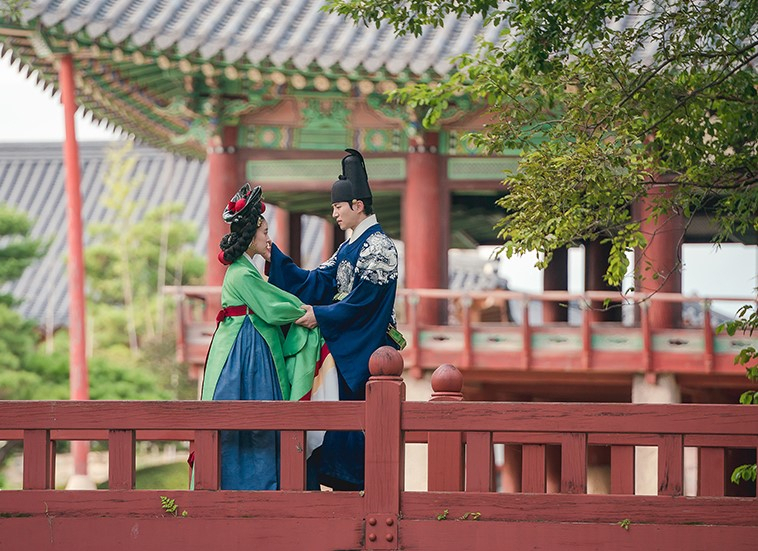The image depicts an outdoor scene in China, featuring a traditional Asian pagoda with reddish wooden columns and a silver, elaborately decorated roof. The background shows a cloudy sky. Slightly left of center, an Asian couple stands facing each other under the pagoda. The woman, who has braided black hair adorned with decorative red ribbons, wears a green robe and a blue skirt, cinched with a red belt. The man, slightly taller, dons a rounded cap with a tiered, longer black cap behind it and is dressed in a dark blue robe with white accents on the shoulders and collar. His left hand holds her arm while his right hand is gently raised towards her face. Behind the couple, there is a red painted wooden railing or bridge, with foliage visible in the upper right corner. The couple appears to share a moment of affection, suggesting they are likely a romantic pair, possibly boyfriend and girlfriend.